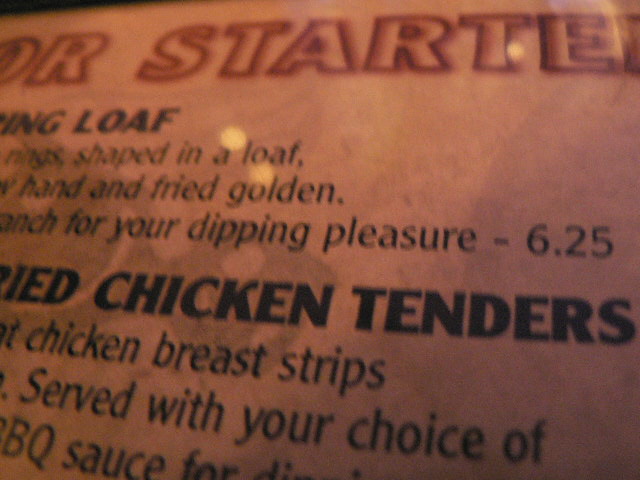This horizontally-oriented color photograph captures a close-up section of a menu under artificial lighting. The image has a yellowish-pinkish tint due to the lighting, which gives it a warm ambiance. The photo, slightly blurry and of lower quality, showcases a menu likely laminated, evident from the light reflections.

At the top of the image, there is an incomplete text within a red outline that appears to say "FOR STARTERS," though the "F" and "RS" are cut off on the sides. Below this heading is the description of a menu item resembling a loaf, described as "fried golden for your dipping pleasure," priced at $6.25. Further down, in large black text, another menu item is listed as "Chicken Tenders." Underneath, a smaller description reads, "Chicken breast strips served with your choice of BBQ sauce."

This snapshot effectively highlights the appetizer section of the menu, despite the slight blurriness and reflections caused by the lighting.